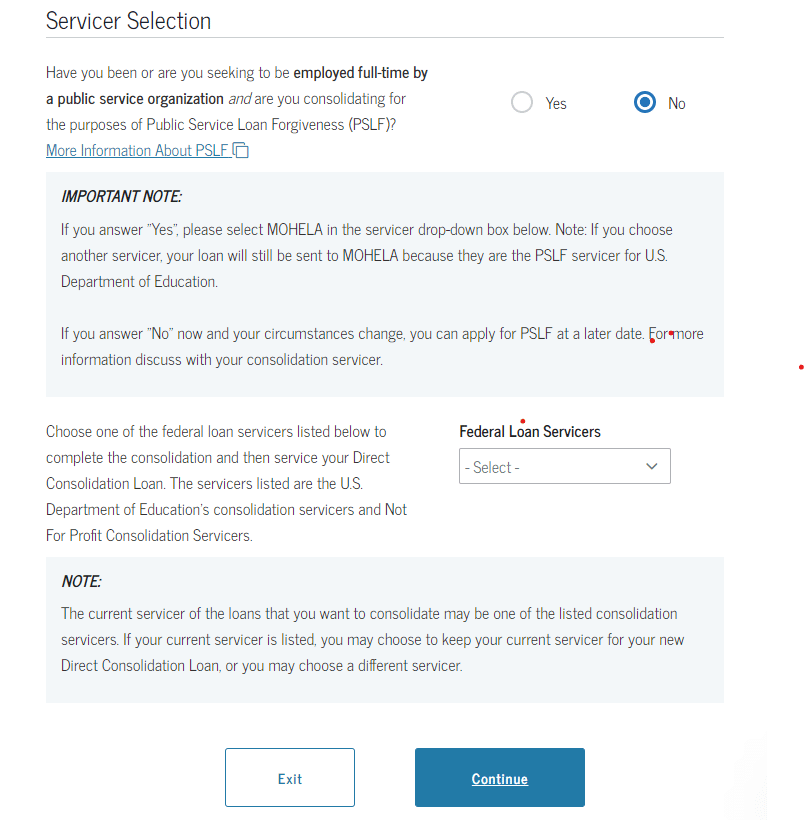### Web Page Screenshot - Loan Consolidation and Public Service Loan Forgiveness (PSLF) Settings

**Background:** White

**Top Left Corner:**
- **Text in Black Font:** "Servicer Selection"

**Below the Title:**
- **Black Horizontal Line:**
- **Instructions in Black Font:** 
  - "Have you been or are you seeking to be employed full-time by a public service organization, and are you consolidating for the purpose of Public Service Loan Forgiveness (PSLF)?"
  - Link to additional information: "More information about PSLF"
  - **Toggle Options:** 
    - "Yes"
    - "No"

**User Interaction Example:**
- **Action Taken:** Click "No"

**Below the Toggle Options:**
- **Important Note:**
  - "If you answer 'Yes', please select 'Mohela' in the servicer drop-down box below. Note: If you choose another servicer, your loan will still be sent to Mohela because they are the PSLF servicer for the U.S. Department of Education. If you answer 'No' now and your circumstances change, you can apply for PSLF at a later date. For more information, discuss with your consolidation servicer."

**Next Section:**
- **Instructions:**
  - "Choose one of the federal loan servicers listed below to complete the consolidation and then service your Direct Consolidation Loan. The servicers listed are the U.S. Department of Education's consolidation servicers and not-for-profit consolidation servicers."

**List of Federal Loan Servicers:** (Details not visible in the screenshot)

---

This revised and detailed caption accurately describes the content and layout of the web page, providing clear instructions and highlighting key points about loan consolidation and PSLF.